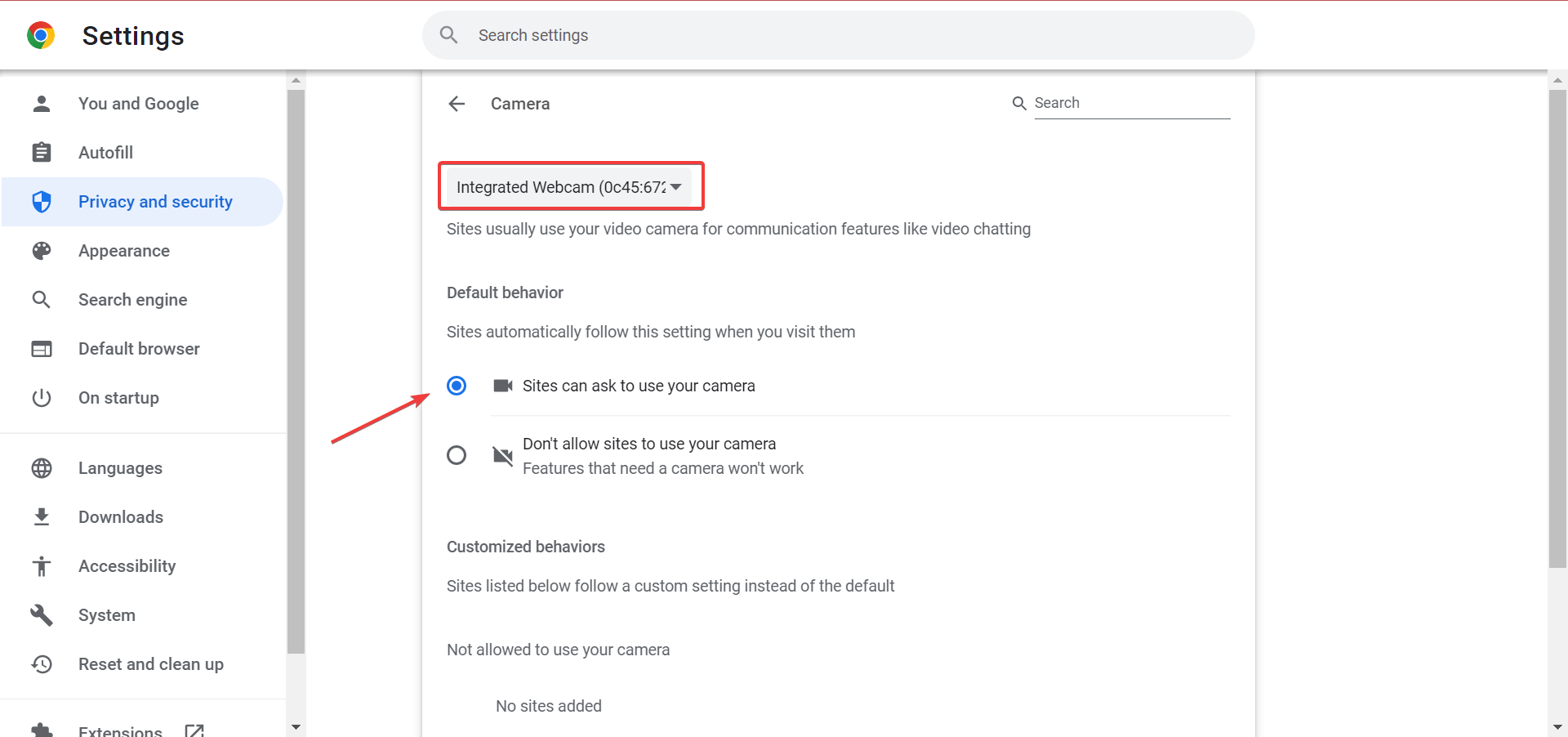The image captures a computer screen displaying a settings page within a web browser. At the top of the screen, a settings menu is visible. Along the left side, a vertical sidebar menu lists multiple categories: starting with "You and Google" at the top, followed by "Autofill," "Privacy and Security," "Appearance," "Search Engine," "Default Browser," and further down, "On Startup."

Continuing down the sidebar, the menu includes "Languages," "Downloads," "Accessibility," "System," and "Reset and Cleanup." Although the lower portion of the sidebar is slightly cut off, a scrollbar is present, indicating that additional options such as "Extensions" are accessible via scrolling.

In the center of the screen, a red arrow points to a specific setting labeled "Sites Can Ask to Use Your Camera." Additionally, a red rectangular box highlights the "Integrated Webcam" setting near the top of this section. This setting features a dropdown menu.